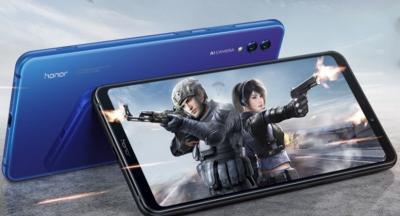In the image, two smartphones are propped against each other on a granite or marble countertop, forming a shape reminiscent of a teepee. The phone in the background, displaying a dark blue back cover, supports the second phone, which is laid out horizontally with its screen visible. This screen portrays a dynamic action scene, likely an advertisement for an action movie or video game resembling "Call of Duty." The vivid depiction shows a paramilitary man and woman, both firing guns with flames erupting from the barrels. The male character, dressed in a blue uniform and wearing a helmet, is on the left, while the female character, clad in a black uniform and a headset, is on the right. Both wield their weapons against a dark, dramatic sky with a road in the background, creating a sense of intense, high-stakes action. The characters appear to extend beyond the phone's borders, adding to the visual impact.